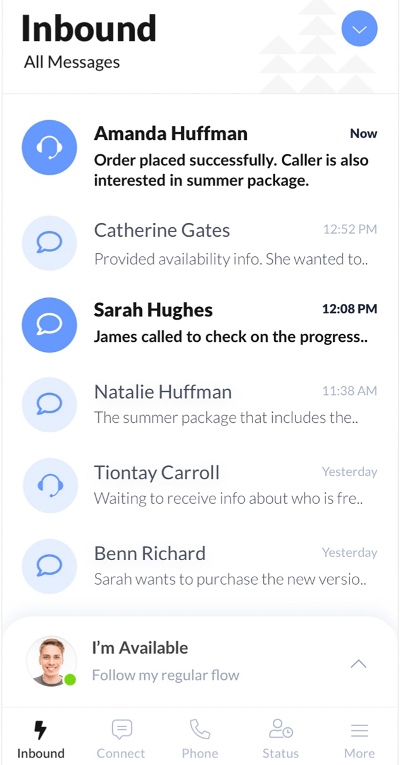This image is a mobile screenshot of a messaging app interface, showcasing an "Inbound" messages section.

At the top of the screen, in bold black font, is the word "Inbound," followed by "All Messages" in a lighter font just beneath it. The top right corner features a dropdown arrow—a white downward-facing arrow set inside a blue circle.

Below this header is a list of correspondents, each with distinct icons indicating types of communication. The topmost entry is for Amanda Huffman, marked with a blue button depicting a white headset, suggesting a phone call. Her message reads, "Order placed successfully," with an additional note mentioning Taylor's interest in her package, and appears to have just arrived.

Next is Catherine Gates, whose icon is a light circle with a blue speech bubble, signaling a text message. Her message, "Provided availability info. She wanted to..." remains truncated with ellipses, received at 12:52 PM.

Sarah Hughes' entry shows an unopened message, indicated by a dark blue button featuring a white speech bubble. Her preview reads, "James called to check on the progress, ..." at 12:08 PM.

Subsequent entries display messages that have already been opened:
- Natalie Huffman's message, received at 11:38 AM, reads, "The summer package that includes..."
- Tyante Carroll has a speaker icon, noting, "Waiting to receive info about who is free yesterday."
- Ben Richard's light blue speech icon accompanies the message, "Sarah wants to purchase the new version that came in yesterday."

Positioned in the lower section is the profile of the app's user—depicted as having fair skin and hair—with a green dot indicating availability. The status reads, "I'm available. Follow my regular flow."

At the bottom of the screen is a navigation bar containing icons labeled as follows: a lightning bolt (Inbound), a speech bubble (Connect), a phone icon (Phone), a clock (Status), and three horizontal lines (More).